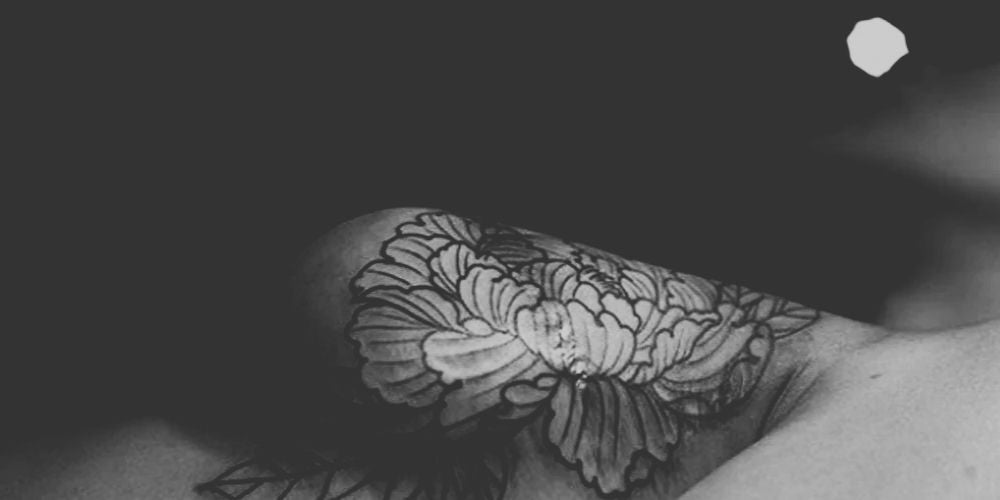The image is a close-up of a black and white tattoo on someone's body, most likely the thigh, though the precise location is difficult to determine due to the zoomed-in nature of the shot. The tattoo prominently features intricate floral and greenery designs, resembling a head of cabbage or lettuce with highly detailed lines and ridges on the leaves. The leaves appear to radiate outward from a central point, with the center having a lighter appearance while the outer leaves are darker. The overall background is predominantly black with shadowed areas of the person's body visible, creating a stark contrast that emphasizes the detailed tattoo. The image is clear and well-lit, devoid of text or numbers, conveying a night-time or somewhat gloomy atmosphere through its monochromatic color scheme.